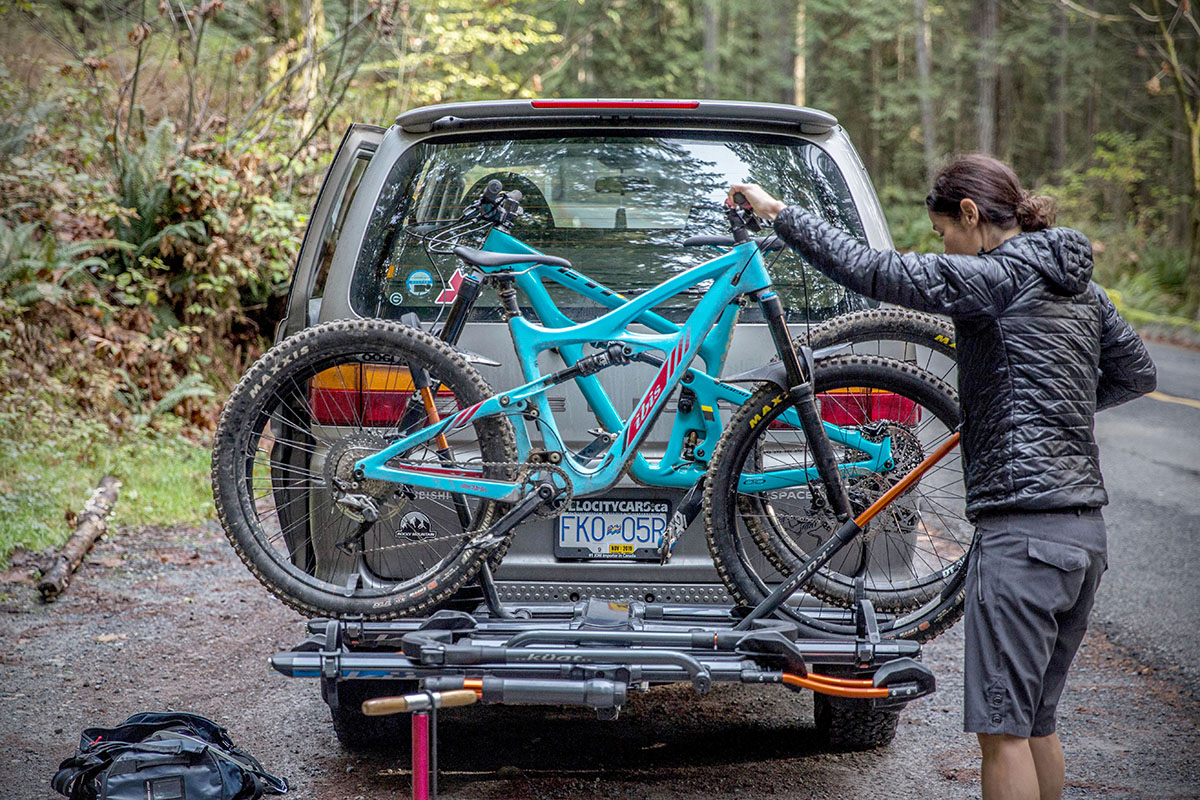In this outdoor daytime photograph, a woman stands behind a gray SUV parked on a roadside bordered by trees and bushes. She is securing one of two teal blue bicycles attached to a bike rack mounted on the vehicle's rear. The woman, viewed from behind, has dark brown hair tied back in a bun and is dressed in a black quilted hooded jacket along with gray cargo shorts that reach her knees. The bike rack, holding two bicycles, is fixed to the SUV’s hitch. On the sandy ground beside the SUV's driver-side rear, a blue backpack and a pink bicycle pump with a light brown handle can be seen. She appears to be either preparing for or concluding a bike ride, with the scene suggesting a tranquil, forested roadside setting.